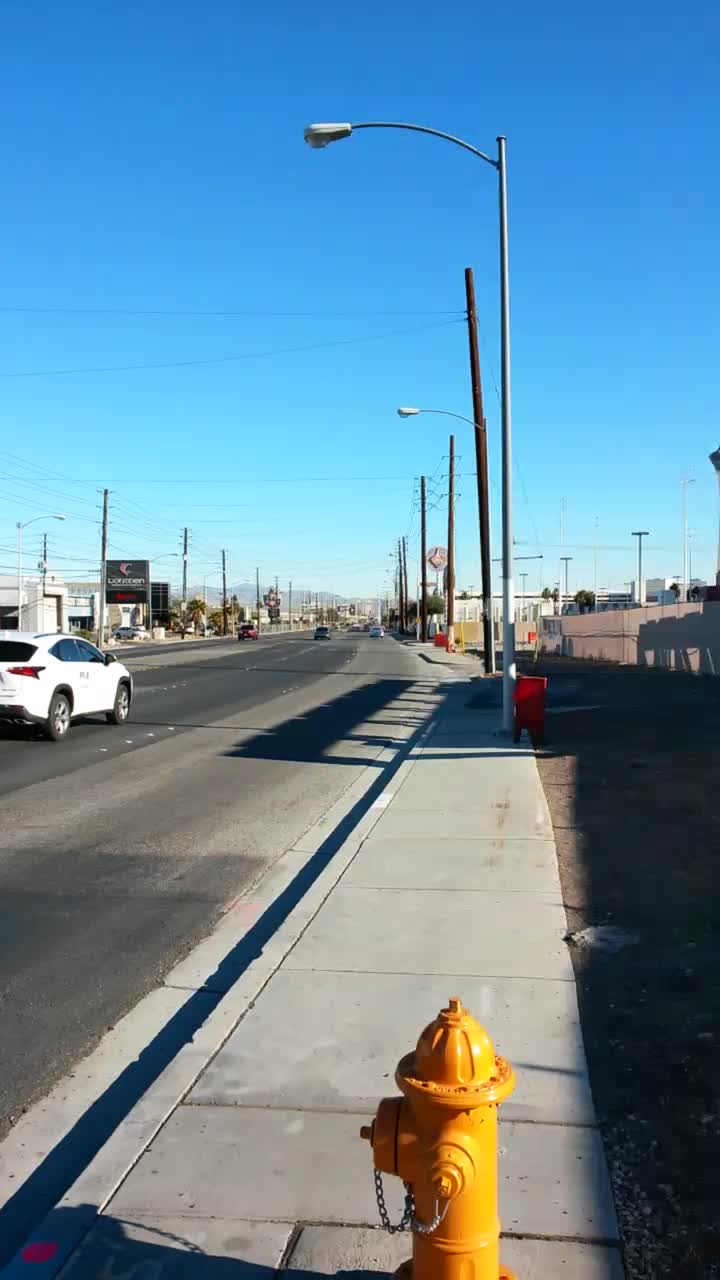This photograph captures a desolate, urban street scene with notable details. The central focus at the bottom of the image is a bright yellow fire hydrant casting a leftward shadow, indicating the sun is shining from the right. The hydrant is situated on a white cement sidewalk that stretches into the distance, flanked on the right by dirt and a tall privacy fence, approximately six to eight feet high. The sidewalk is dotted with utility poles, some connected to wiring and some not, and a single silver-gray street light that arches over the roadway. On the left side of the street, a white car, possibly an SUV, drives from the center-left towards the center of the image. This road appears to have multiple lanes, potentially four to six, with more utility poles and light poles lining its edges. In the background, businesses line the far side of the street, while the horizon fades into a distant mountain and a pale blue sky overhead. The overall atmosphere is one of urban decay, with a notable amount of rubble and a somewhat deserted look.